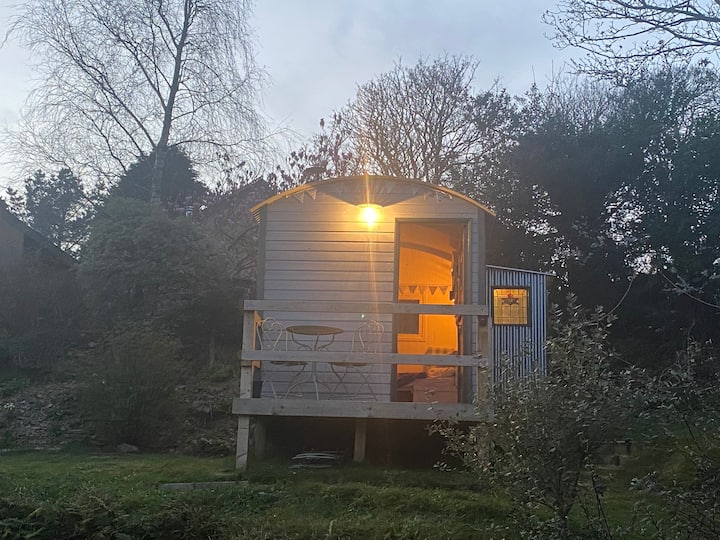This photograph, taken during the crepuscular hours when the sky retains a deep blue hue, showcases a small, minimalistic mobile home nestled in a forested area. The mobile home, elevated on stilts without a visible foundation, features a rounded roof and is flanked by dense trees, some of which are barren, hinting at the winter season. A tiny, weather-worn deck juts out from the front, supporting a modest table and two metal chairs, welcoming visitors to sit and enjoy the serene environment. The open door and illuminated porch light, glowing a strong yellow, shed a warm, orange light within, revealing glimpses of the compact, cozy interior. Additional details include a small shed attached to the side of the home and lawn chairs tucked neatly under the deck. The entire scene is bathed in the calm, dim light of either early evening or morning, capturing the tranquil atmosphere of this tiny woodland retreat.